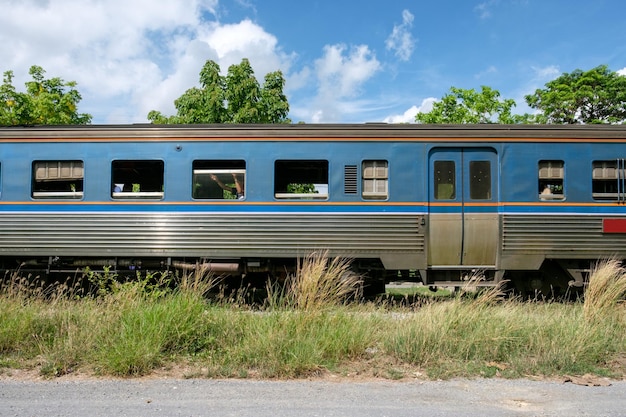This detailed photograph captures a single section of a vintage, blue railway passenger car on a calm day, presumably stopped on the tracks, surrounded by a serene landscape. The sky above is a crisp blue adorned with white, fluffy clouds. The railcar, featuring an orange stripe running horizontally along its blue and unpainted steel sides, is centrally framed in the image, drawing attention to its old-world charm. A close look reveals several windows along the side of the train; some are open, with a noticeable individual seen lifting one window, suggesting the train is still in use. In the foreground, there's a stretch of unkempt grass and a dirt road leading towards the railcar, with a backdrop of lush green trees completing the scene. The composition and clarity of the image suggest that the train may be at a standstill, providing a nostalgic glimpse of travel from a bygone era.